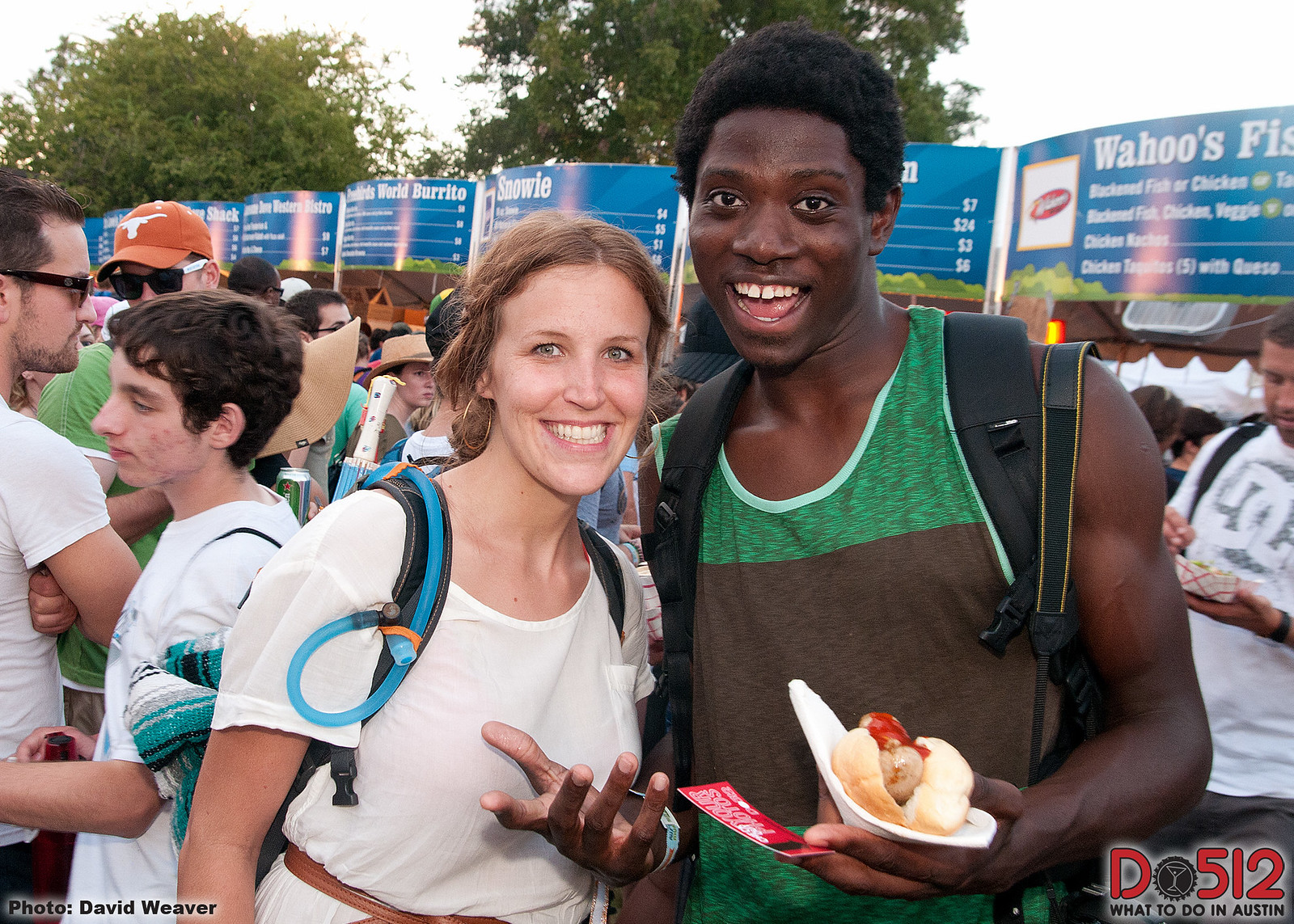The image captures a lively outdoor festival in Austin, Texas, indicated by a watermark in the lower right corner that reads "D, circle 512" and "What to Do in Austin." In the foreground, a smiling woman with brown hair tied back stands on the left. She wears a white t-shirt with a left chest pocket, a brown belt, hoop earrings, and carries a backpack with a noticeable blue drinking tube. Next to her, on the right, stands a smiling man, an African American with black hair, donning a green and brown tank top. He holds a paper plate with a hot dog or bratwurst in his left hand, along with a red ticket stub and a white napkin. A blue paper bracelet is visible around his right wrist. The man also wears a black backpack. The background is bustling with casually dressed festival-goers and features trees and various food vendor stalls, including signs for "Western Bistro," "World Burrito," and "Wahoo's Fish," which offers items like blackened fish, chicken, and veggie options, chicken nachos, and chicken taquitos. The lower left corner of the photograph credits David Weaver as the photographer.